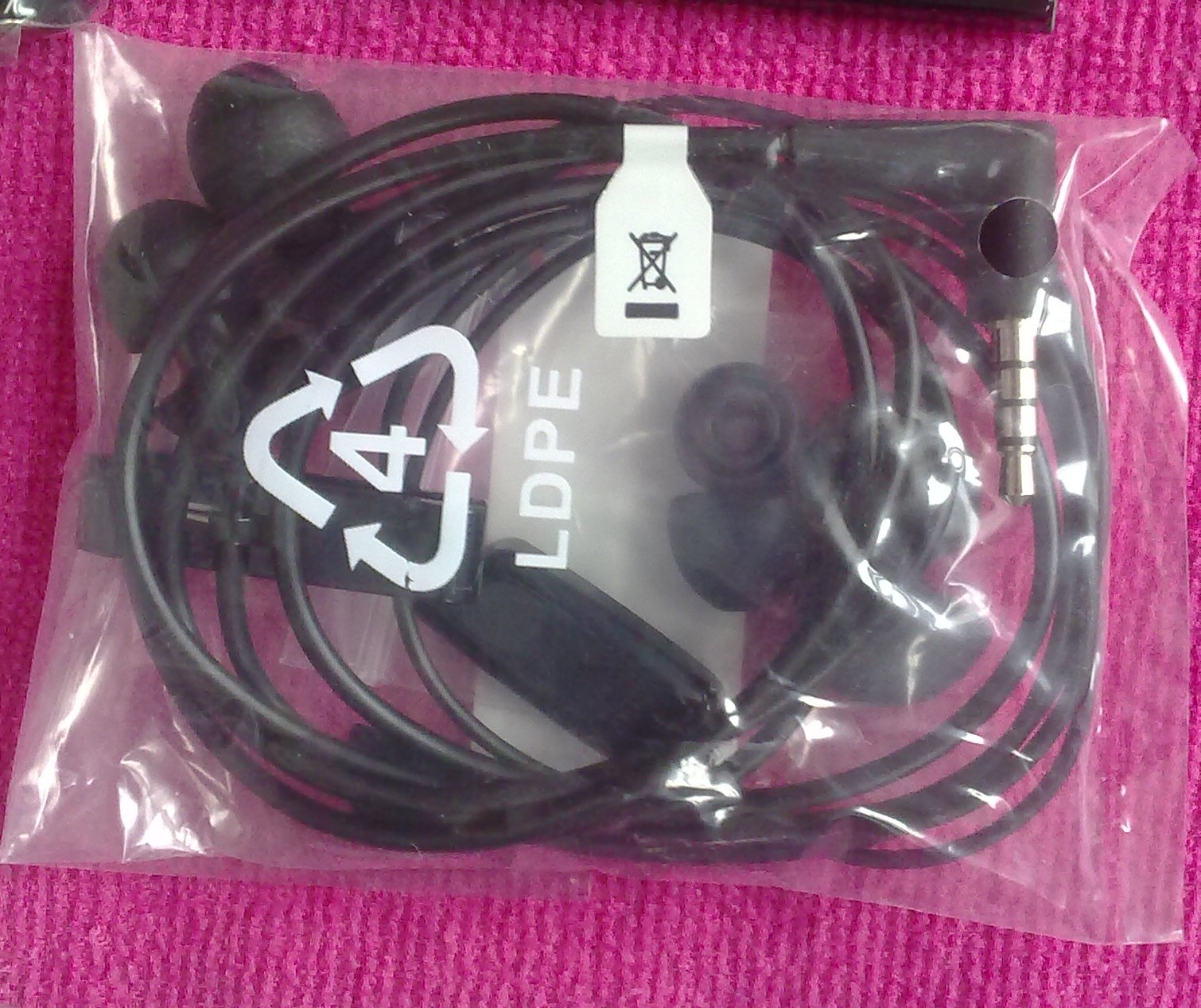The image is an up-close, color snapshot photograph taken with a flash, showcasing a pair of in-the-ear earbud headphones wrapped in their original clear plastic packaging. The headphones feature a long, coiled cable with a headphone jack and two spare silicone earpieces included inside the see-through bag. The packaging is heat-sealed at one end and folded over at the top, secured with a bit of sellotape. Prominent on the bag are recycling symbols, including a "4LDPE" logo with arrows and a sticker depicting a crossed-out wheelie bin, signalling not to dispose of it in regular trash. The cable also has a small tag bearing this caution. The entire package rests on a vibrant, flamingo-pink, fuzzy fabric, which could be a carpet or a blanket, highlighted by the camera’s flash.